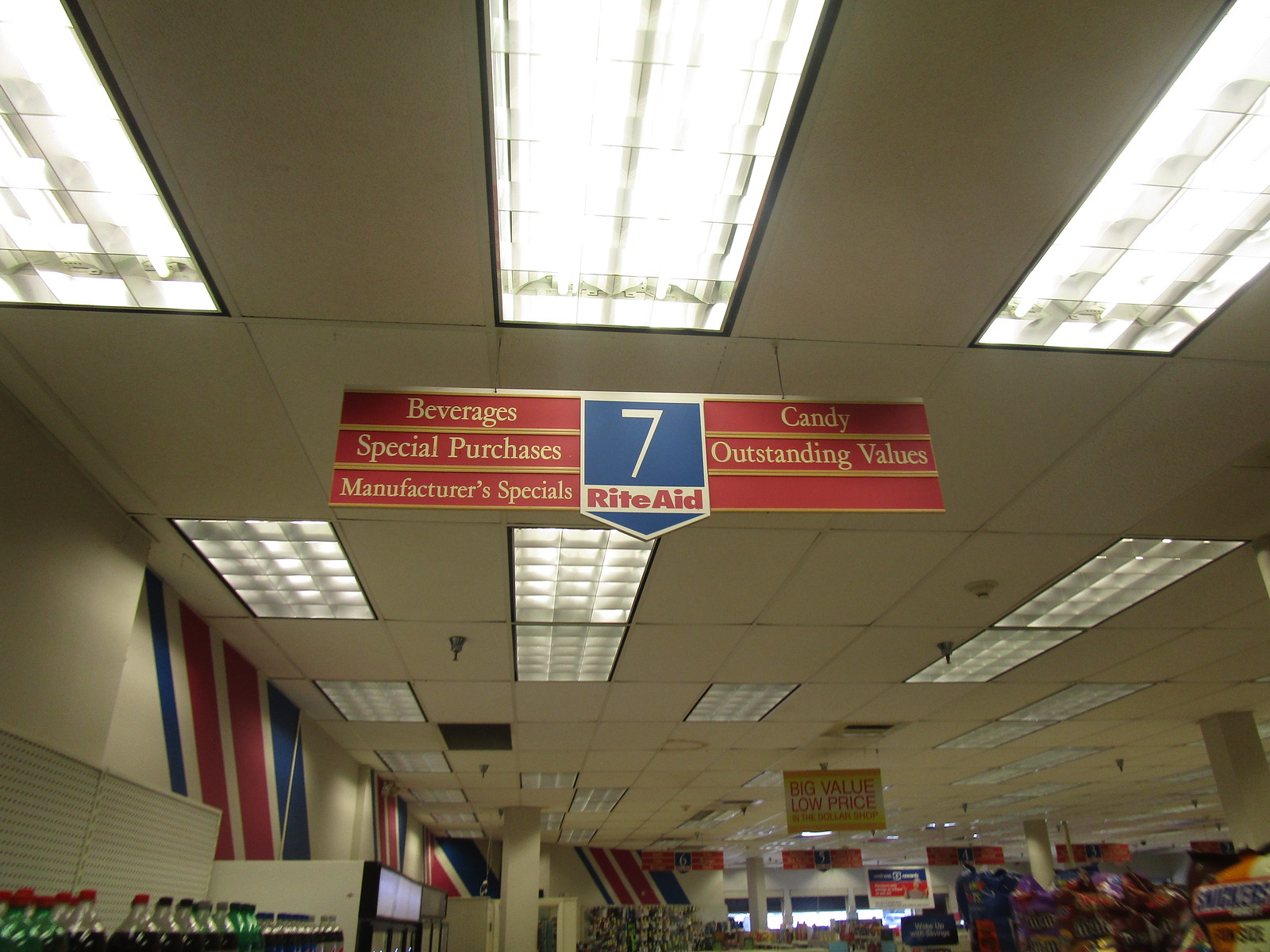A detailed view inside a bustling store reveals a distinct light brown ceiling adorned with numerous large ceiling lights that illuminate the space. Dominating the scene is a prominent sign suspended in the middle of the store. This eye-catching sign is primarily blue and shaped like a shield, featuring a central gray number 7. A gray strip runs across the middle of the sign, proudly displaying the words "Rite Aid" in bold red letters. The bottom of the shield is blue, bordered with a gray outline.

Flanking this central sign are additional signs in red, each inscribed with gold letters. These signs direct shoppers to various sections of the store, including "Beverages," "Special Purchases," "Manufacturer Specials," "Candy," and "Outstanding Values." The walls are decorated with vibrant red and blue stripes that add a lively touch to the store’s interior.

The store is well-stocked with a variety of products; prominent displays of TV sets and stacks of Snickers bars can be seen among an array of other items, creating a vibrant and busy atmosphere that caters to a wide range of shopper needs.